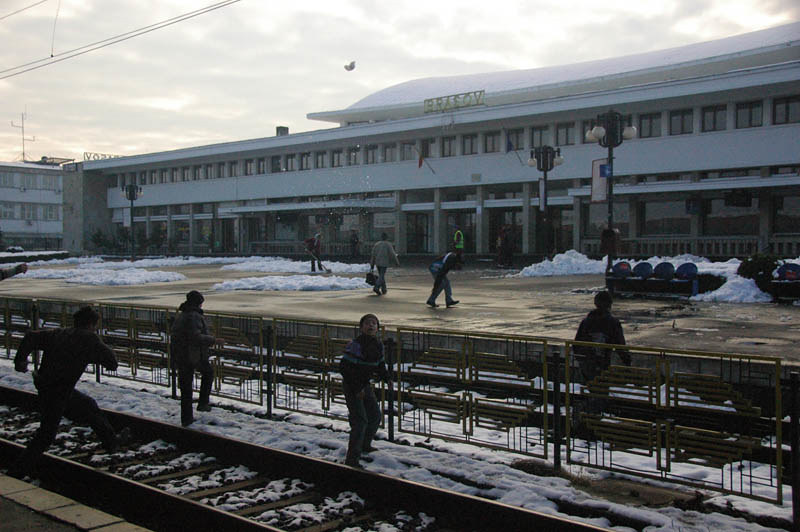The photograph captures an outdoor scene at a train station, likely during dusk or dawn given the dim, overcast sky with some sunlight trying to peek through. The station's main building is predominantly white with gray accents and stretches from the left side of the image to the right, partially cropped out. The building is substantial in size, at least two stories tall, and features numerous windows, which could hint at some level of elegance or age. Above the main entrance, golden lettering, possibly in Cyrillic or Greek, spells out "Brazov." 

In the foreground, a set of train tracks extends from the bottom left towards the bottom center of the image. Parallel to these, a golden railing runs horizontally across the center, obscuring a second set of train tracks in the background. The tracks and the railing appear beige or rusted, suggesting some age or wear. Snow is scattered throughout, lightly covering parts of the tracks and the ground, gathered in little mounds, except on the railing. The ground itself is a dark brown concrete.

In the midst of this snowy setting, four young boys are playing on the tracks. Three of them are close to the central railing, seemingly in motion and about to cross over. One boy at the center looks directly at the camera, while the other two are mid-crossing. To the left, a cropped-out hand hints at another child nearby. On the other side of the railing, at the back set of tracks, stands another boy who has already crossed.

The scene is vibrant with activity: adults and children move about the courtyard area in front of the train station, where little mounds of snow are scattered. Towards the center-left in the background, someone can be seen shoveling snow. Streetlights and dark blue benches dot the area, adding to the station’s functional aesthetics. Overall, the image presents a lively yet serene winter day at a bustling train station, with a hint of historical elegance in its architecture.